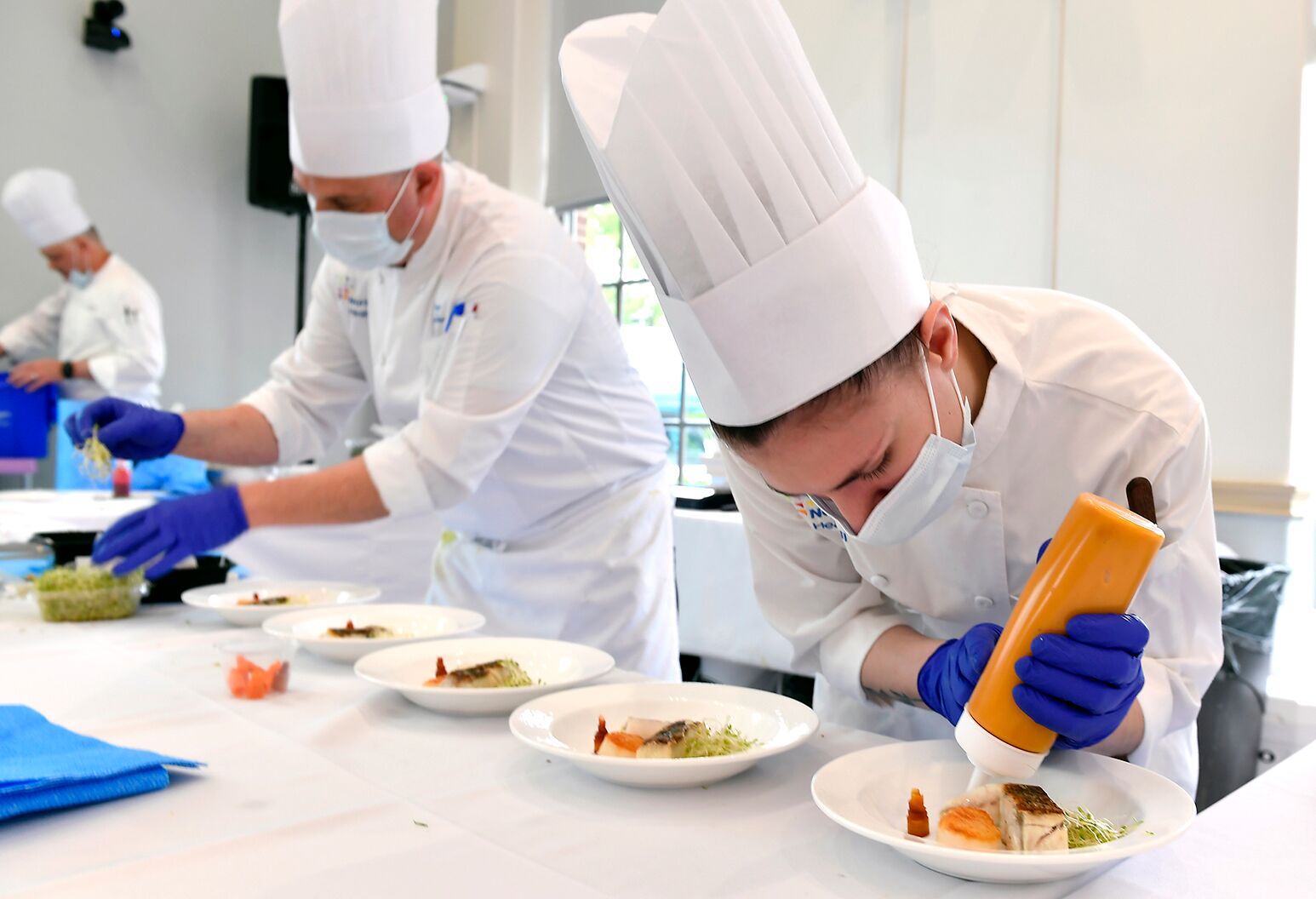This photograph depicts a trio of chefs meticulously preparing dishes at a long, white table, possibly in a professional kitchen or culinary school setting. All three chefs are fully dressed in traditional chef's uniforms, complete with tall white hats, white aprons, and blue latex gloves. They are also wearing masks, emphasizing a hygiene-centric environment. The scene appears to be organized like an assembly line, with each chef contributing to the completion of gourmet meals.

In the foreground, a female chef, focused and precise, is holding an orange squeezable bottle upside down, adding a sauce to a white plate. Beside her, a male chef, also in white attire and purple gloves, is carefully placing greenery embellishments on the dishes. The plates, possibly holding delicacies like fish or oysters, are arranged in a row, demonstrating the systematic nature of their task. In the background, another chef, wearing a blue mask under his chin, is working at a separate station, contributing to the collective effort. Blue napkins and neatly aligned bowls or plates enhance the neat and orderly appearance of this culinary workspace, hinting that the team is prepping for a restaurant's night service.